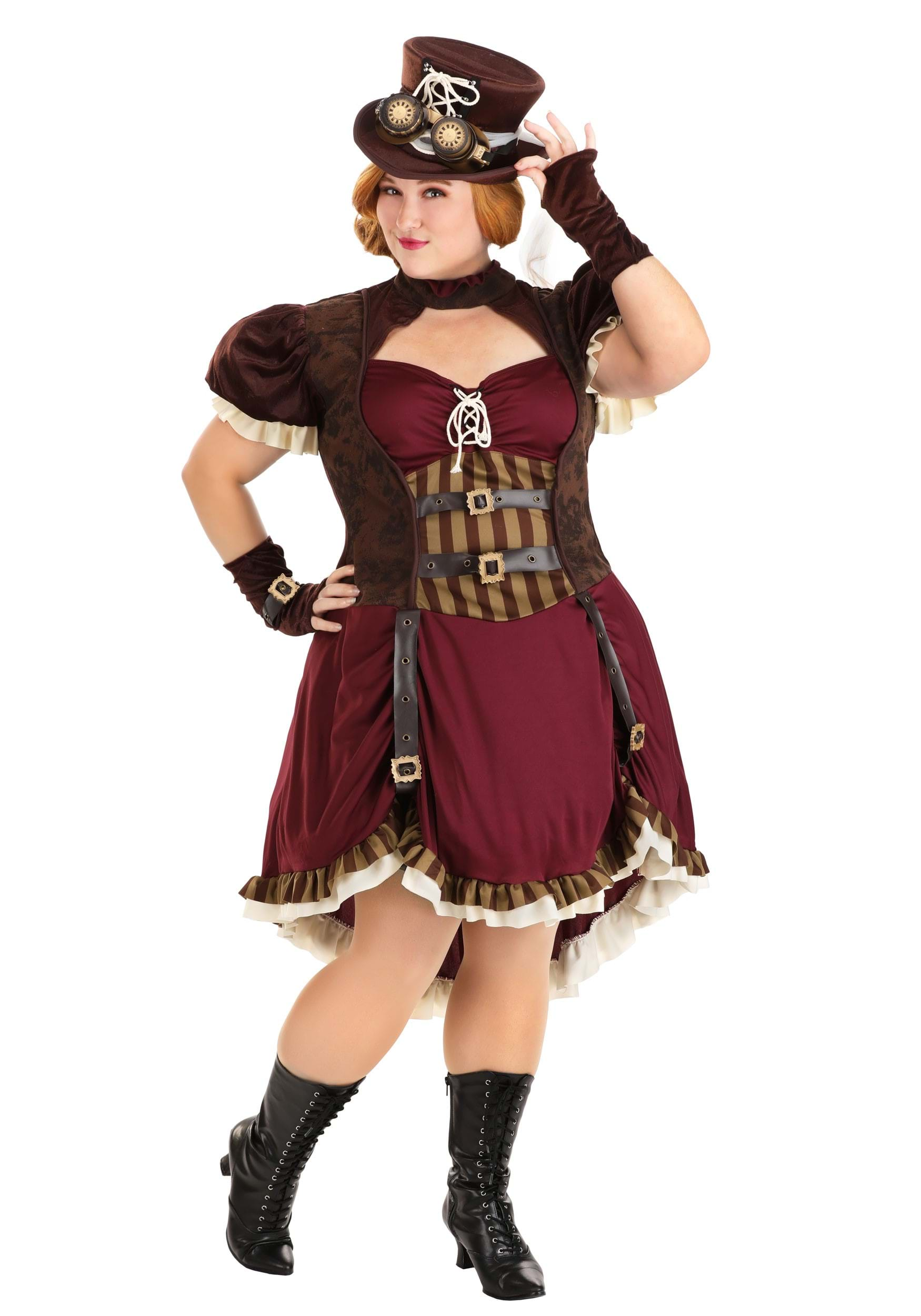In this image, we see a young Caucasian woman cosplaying in a steampunk-inspired outfit, set against a pure white background. She is wearing a burgundy dress that features prominent steampunk elements. The dress has white ruffled trim at the bottom and sleeves that extend just past her elbows. Leather straps with gold buckles run vertically down the dress, and there's a garter area with additional horizontal leather straps and gold clasps. The upper part of the dress includes white lacing over the breast area. Accompanying the dress is a matching burgundy jacket.

Her accessories enhance the steampunk aesthetic: she sports black leather, heeled boots that lace up from the toes to midway up her calves, and fingerless brown gloves. Topping off her ensemble, she wears a dark reddish-purple, almost burgundy fedora adorned with a white ribbon and white strings tied in a bow, which sits above ginger-colored, short, wavy hair that reaches her ears. Additionally, gold-colored goggles rest on top of her hat.

The combination of these intricate details makes for a striking and cohesive steampunk cosplay, showcased clearly for all to see against the background.